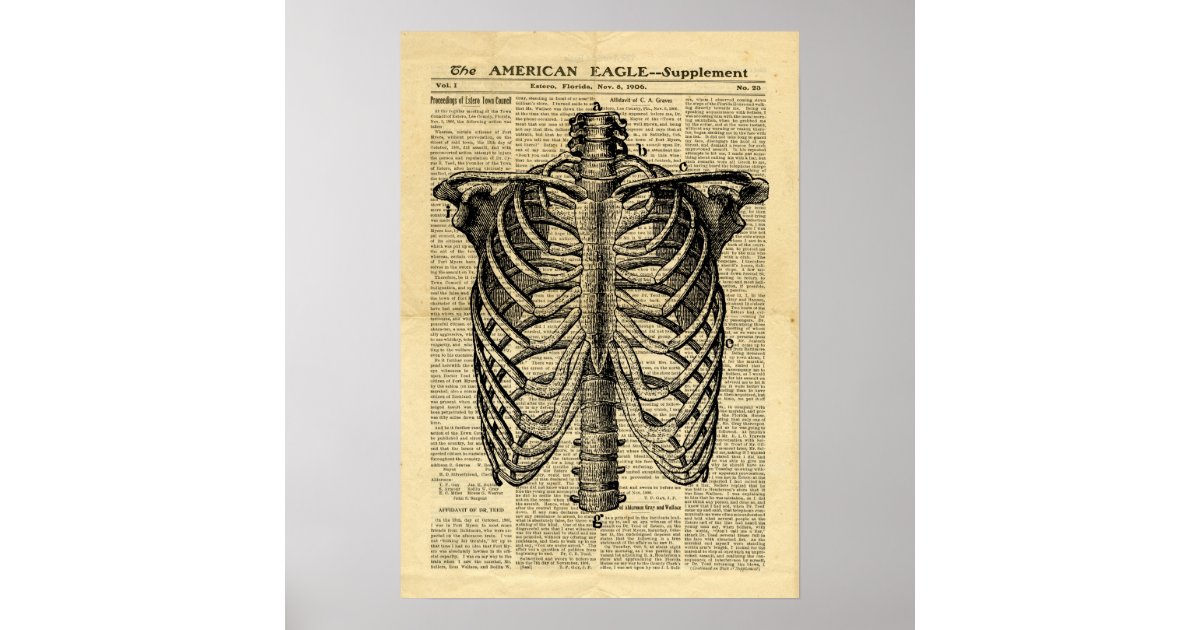This composite image features two distinct subjects. The first is a newspaper article from "The American Eagle," specifically a supplement published in Estero, Florida, on November 8th, 1906 (Volume 1, Number 28). The headline reads "Proceedings of Estero Town Council." The article is set against a light gray background.

Superimposed over the newspaper article is a detailed drawing of a human skeletal rib cage and part of the spinal column. The illustration is annotated with letters (A, B, C, G, and J) to identify specific portions of the skeleton. This skeletal drawing is precisely centered on top of the newspaper, creating a striking and informative visual contrast.